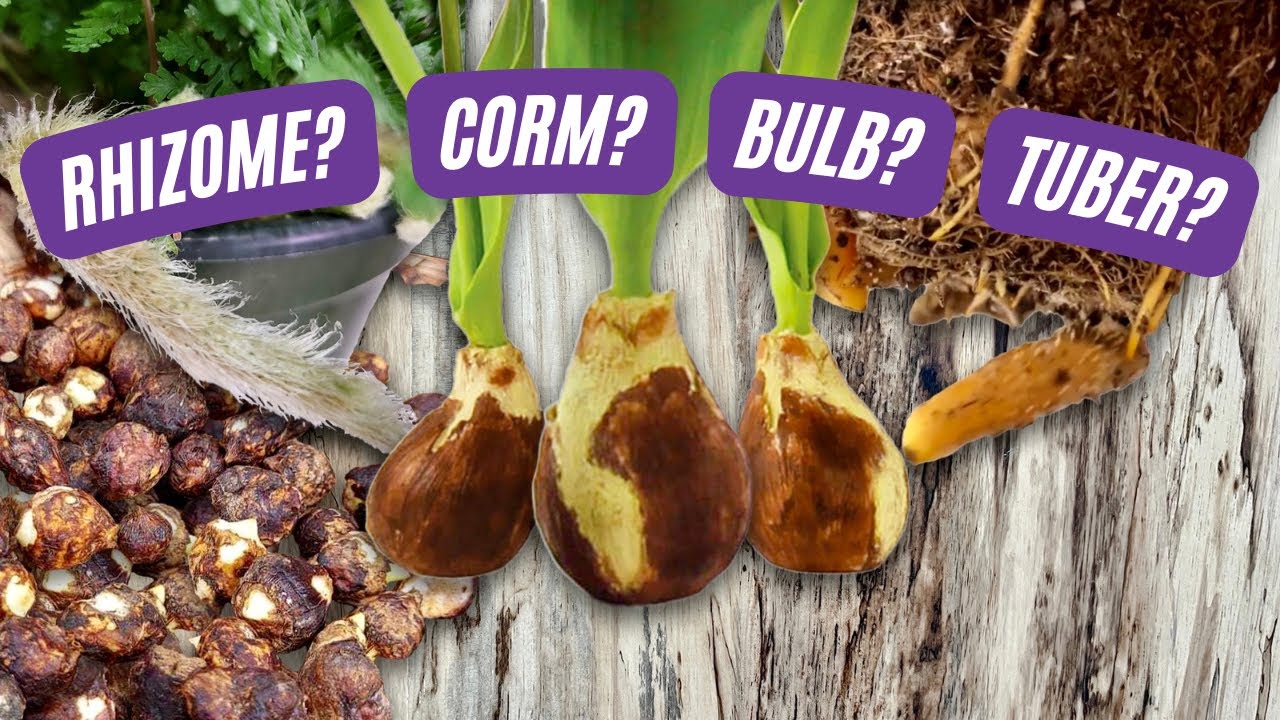The image displays a collection of various plant parts arranged on what appears to be a worn, faded tree bark background. Prominently featured in the center are three bulbous plants with brown and beige tones, each sprouting green stems and leaves. Surrounding these central bulbs are different types of plant structures, each labeled with a purple rectangular text bubble with white writing. The labels read "RHIZOME?", "CORM?", "BULB?", and "TUBER?". The top left corner shows green leaves, while the top right reveals a tangle of dark brown, root-like forms. In the bottom left, there is a cluster of small, dark brown objects that could be either nuts or small vegetables. The various plant parts and their settings create a natural, earthy scene, with emphasis on different types of roots and underground structures for growing plants.